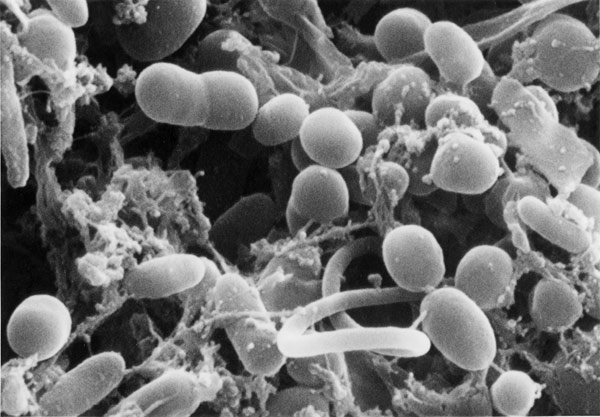The image depicts a black and white, electron microscope view of a microscopic organism, likely bacteria or a virus. The photograph showcases numerous lighter-colored pod or seed-like structures that appear cylindrical and are interspersed with darker, shadowed areas. Connecting these pod-like formations are white, stringy, cobweb-like fibers that weave throughout the image. Toward the lower center, a worm-like structure spirals, adding a dynamic element to the composition. The overall appearance is highly detailed and three-dimensional, reminiscent of medical imaging techniques used to study microscopic life forms.